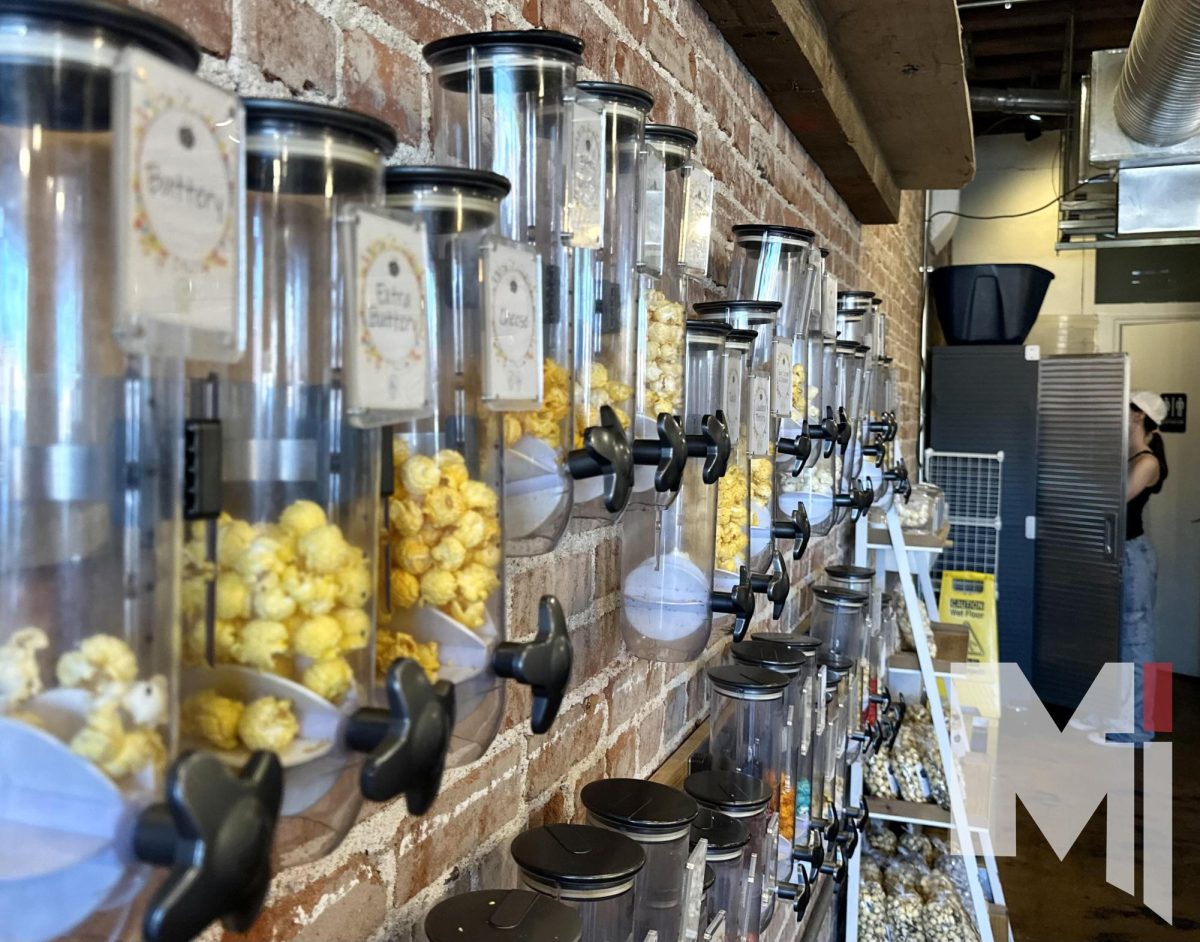This rectangular image, which is wider than it is tall, captures the inside of a gourmet popcorn shop. Along the left side of the image, a brick wall is lined with a series of clear acrylic dispensers, each fitted with black twist knobs. These dispensers, filled with various types of popcorn, are meticulously labeled, with the closest visible labels reading "buttery" and "extra buttery." Beneath these dispensers, additional canisters are visible. Toward the front of the image, there are containers that might hold cookies, candies, or pastries, adding to the shop's assortment. On the right side of the image, a woman wearing a white hat stands near a metal storage unit, appearing to retrieve something from it. The overall scene offers a detailed glimpse into the diverse offerings and setup of the popcorn shop.